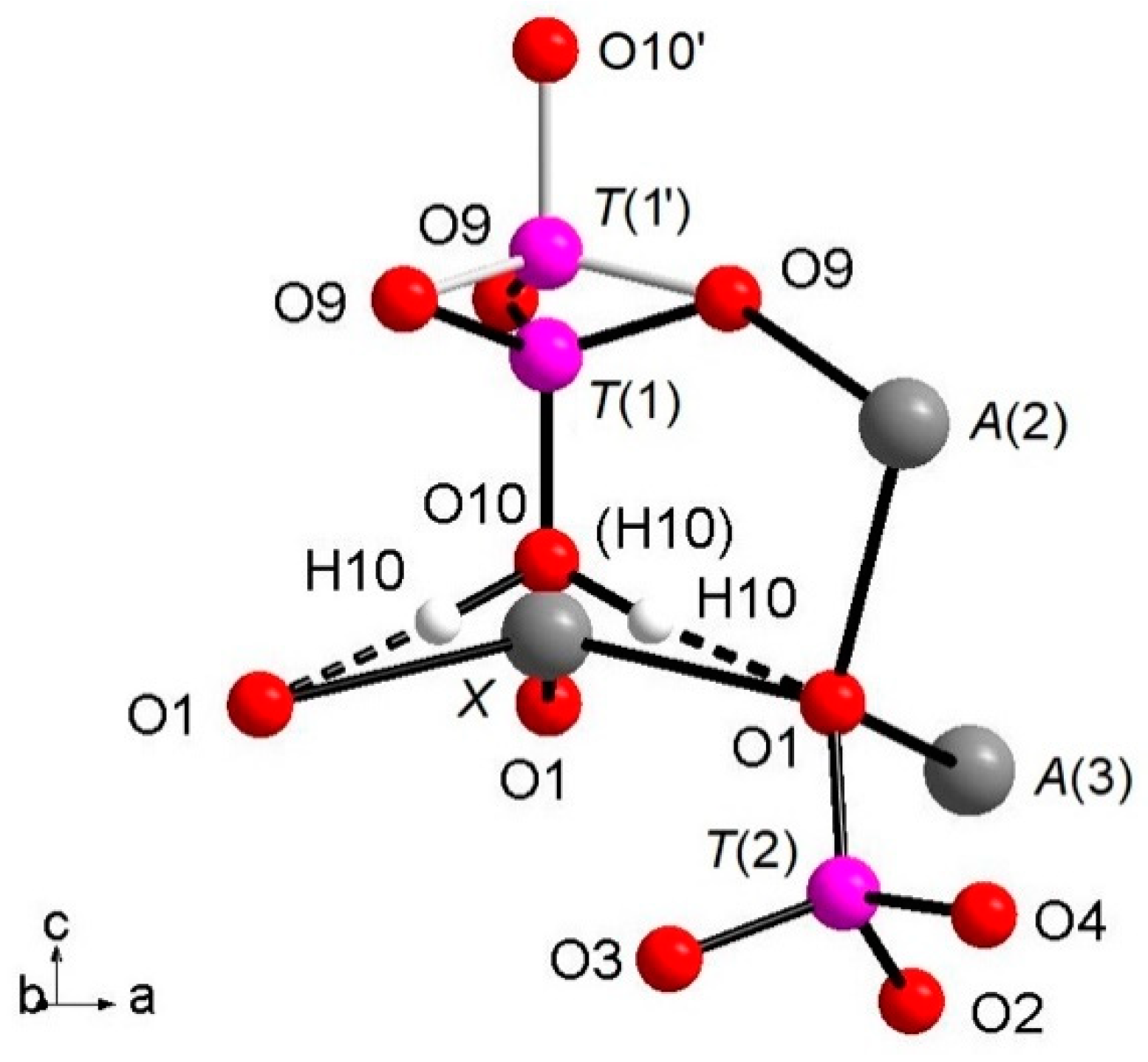The image is a detailed diagram of a molecule, visually represented by various colored balls connected by straight and black lines. The colors used include red, pink, gray, and white, with each ball accompanied by a label specifying different symbols and numbers. At the top of the diagram is a red ball labeled "O10" followed by an apostrophe. A white line descends from this ball to connect with a pink ball labeled "T(1)’," which branches off to three red balls labeled "O9." Other parts of the diagram feature additional red, gray, and white balls labeled with various symbols such as "H10" in parentheses, "O3," "O2," "O4," and "A2." In the bottom left corner, the letters A, B, and C are present, connected by arrows pointing left, right, and upward, respectively. Despite the detailed labeling, no title or explanatory text is provided, making it reminiscent of something typically found in a chemistry textbook.